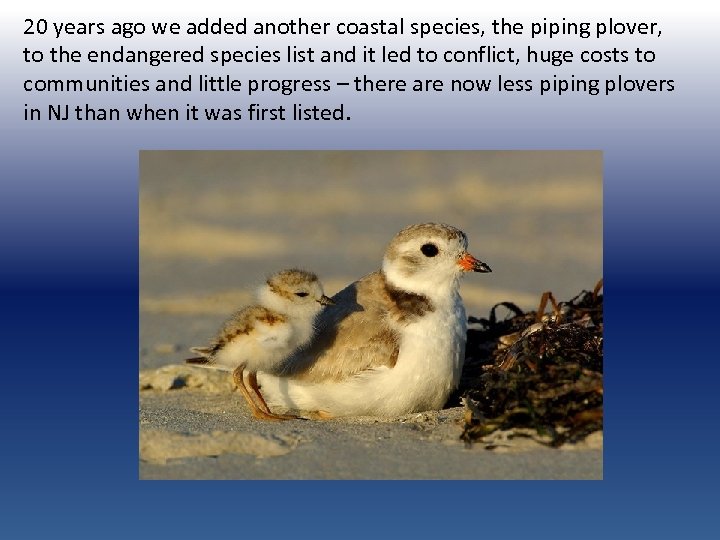The image is an educational slide featuring a central photograph of two piping plovers, a mother and her chick, situated on a sandy area near some dark brown seaweed or vegetation. Both birds are depicted in profile, looking to the right; the mother is sitting while the chick stands close in front of her. The birds are characterized by their white undersides, light brown tops, orange beaks, and dark black eyes. The slide's background is a gradient ranging from white to dark blue to lighter blue, and it contains a sans-serif font text at the top. The text reads: "Twenty years ago, we added another coastal species, the piping plover, to the endangered species list, and it led to conflict, huge costs to communities, and little progress. There are now fewer piping plovers in NJ, New Jersey, than when it was first listed."